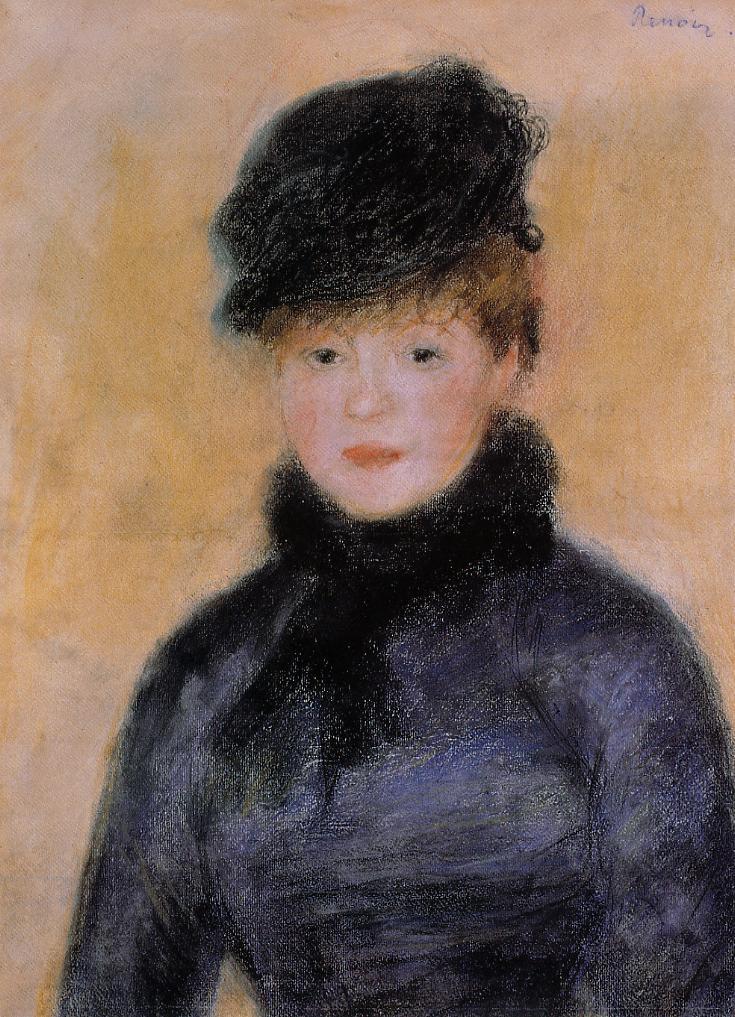This impressionistic portrait painting of a woman, likely inspired by the late 1700s or early 1800s, features a dreamy, almost unfocused style reminiscent of soft pastel drawings. Her face, framed by short, reddish-brown hair and a black fashionable derby-style hat, is rendered with faint, delicate outlines, highlighting her dark, serious eyes, orangish-red lips, and subtly blushed cheeks. She wears a sophisticated black scarf that wraps around her neck and a deep, bluish-gray coat with no discernible buttons or pockets, covering her torso up to her waist. The soft background consists of scribbly, beige, and orange-red hues, adding to the painting's ethereal quality. In the top right corner, the name "Ramon" is inscribed in blue lettering.